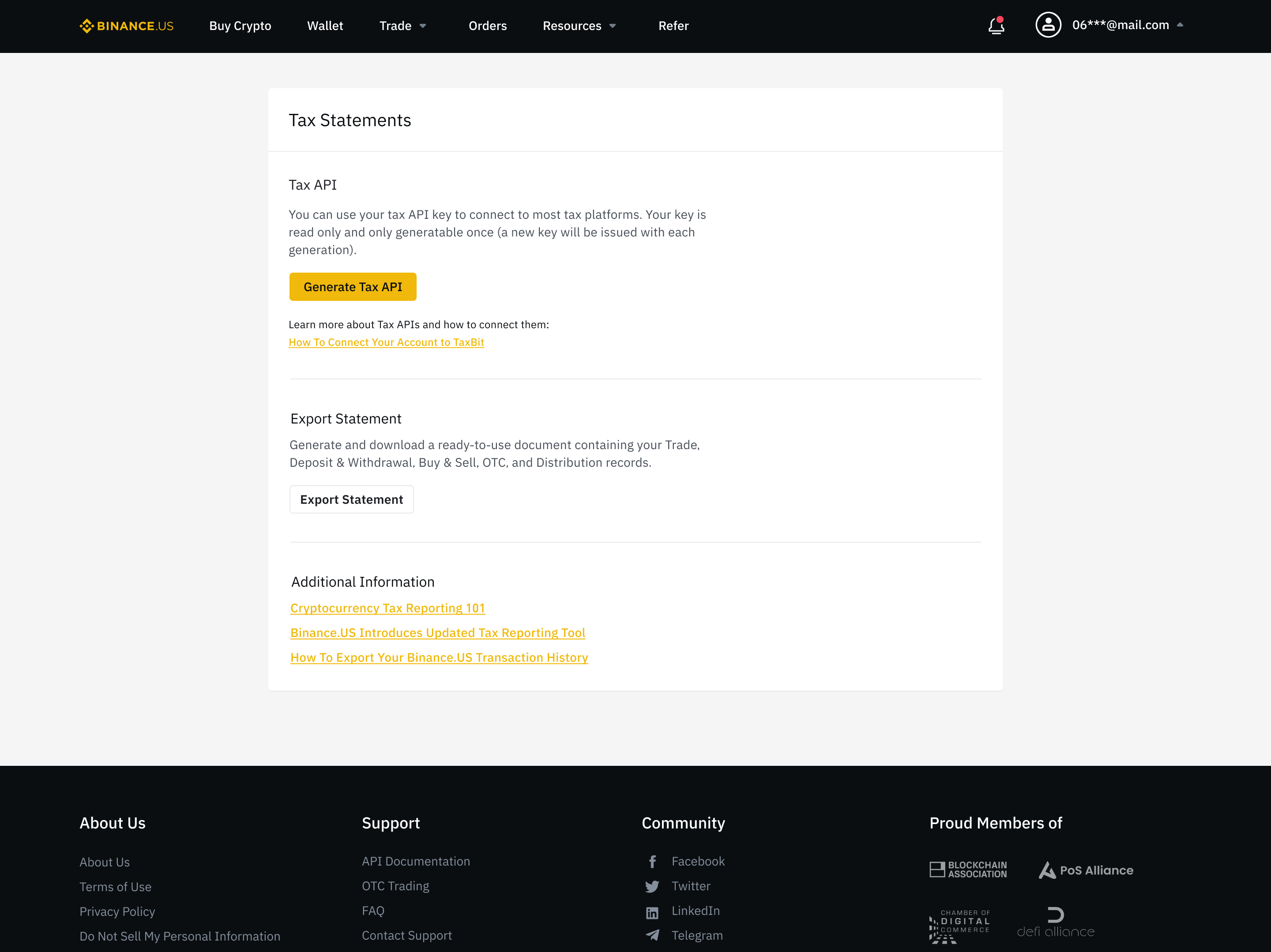This screen capture from the Binance US website showcases the main navigation bar and a tax statement management section. At the top, a black navigation bar features categories such as "Buy Crypto," "Wallet," "Trade," "Orders," "Resources," and "Refer." To the far right, there is a bell icon with a red notification dot, and the user's account name is displayed.

Below the navigation bar, the main content area consists of an off-white square with a prominent white square in the center. This section is titled "Tax Statements" and provides information about using a Tax API key to connect to most tax platforms. The note emphasizes that the API key is read-only and that a new key will be issued with each generation. There is a prominent yellow button labeled "Generate Tax API," along with a hyperlink to learn more about tax APIs and how to connect your account to TaxBit.

Additionally, users can click a yellow button labeled "Export Statement" to generate and download a document containing their trade, deposit, withdrawal, buy, sell, OTC, and distribution records.

At the bottom of the screen, an information section lists three hyperlinks: "Cryptocurrency Tax Reporting 101," "Binance US Introduces Updated Tax Reporting Tool," and "How to Export Your Binance US Transaction History."

The footer of the page is entirely black and includes links for "About Us," "Support," and "Community," along with a note about the company's memberships, though the specific affiliations are not fully visible in this screen capture.